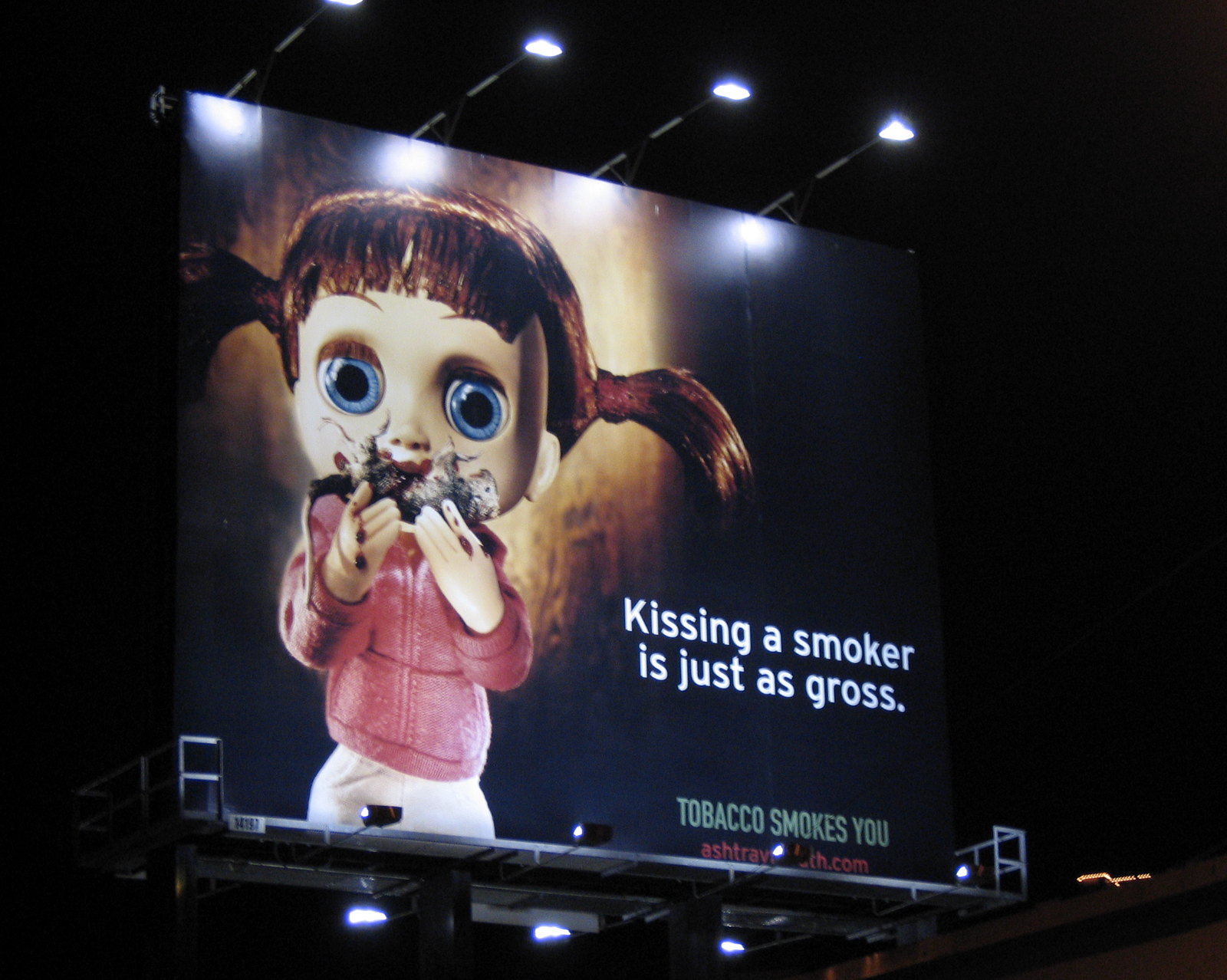This nighttime photograph captures a large rectangular billboard illuminated by four white lights at the top and additional lights at the bottom, creating a dramatic effect. The billboard features an unsettling image of a highly stylized little girl with brown pigtails and large circular blue eyes, widely resembling a doll. She wears a pink hoodie and white pants. Her face, particularly around the mouth, is covered in what appears to be dirt or ash. She holds her hands up to her mouth, with what looks like a dead rat's tail hanging from them, suggesting she might be in the act of eating the rat. To the right of the image, bold white text states, "Kissing a smoker is just as gross." Below that, in green font, it reads, "Tobacco smokes you." The billboard sends a stark anti-smoking message, enhanced by the eerie and disturbing visual elements.